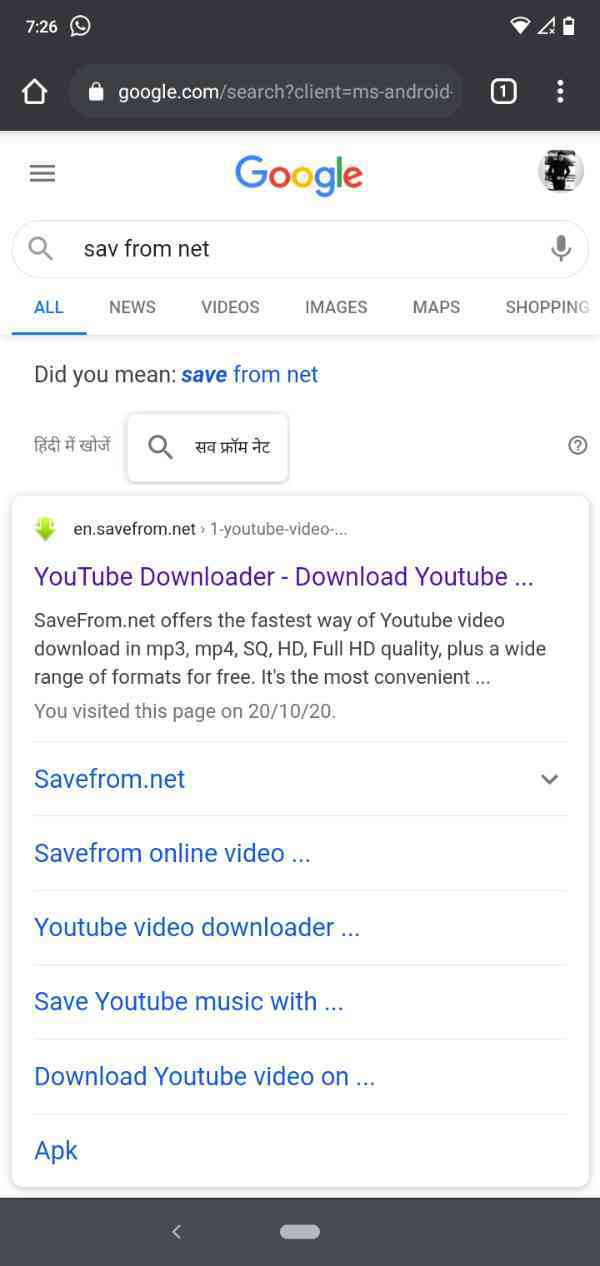This is a detailed caption of an image portraying a cellphone screenshot of a Google search:

In this portrait-oriented cellphone screenshot, the time displayed at the top is 7:26 AM, along with a black bar harboring the address bar, phone, WhatsApp indicators, Wi-Fi status, and battery level. The browser interface indicates this is the only tab open, and there's a menu icon with three dots on the top right. The Google logo in its familiar blue, red, yellow, green, and red hues is prominently featured, with the search query "Sav from Net" entered in the search bar. The search results page is open with the "All" tab highlighted, alongside options like News, Videos, Images, Maps, and Shopping, suggesting the presence of additional tabs.

Underneath the query, Google suggests "Did you mean Save from Net?" and displays text in another language. The first result is a prominently visited link (indicated by its purple color): "Saveform.net," described as a YouTube downloader offering fast downloads in various formats and qualities, including MP3, MP4, SQ, HD, and Full HD, free of charge. The page notes it was visited on October 20, 2010. Below this entry, a dropdown arrow suggests further navigation options.

Additional search results include titles like "Save from Online Video," "YouTube Video Downloader," "Save YouTube Music With," and "Download YouTube Video On," followed by the term "APK." The bottom part of the screen shows the phone's status bar with standard icons, rounded off by a black background typical of most phone interfaces.